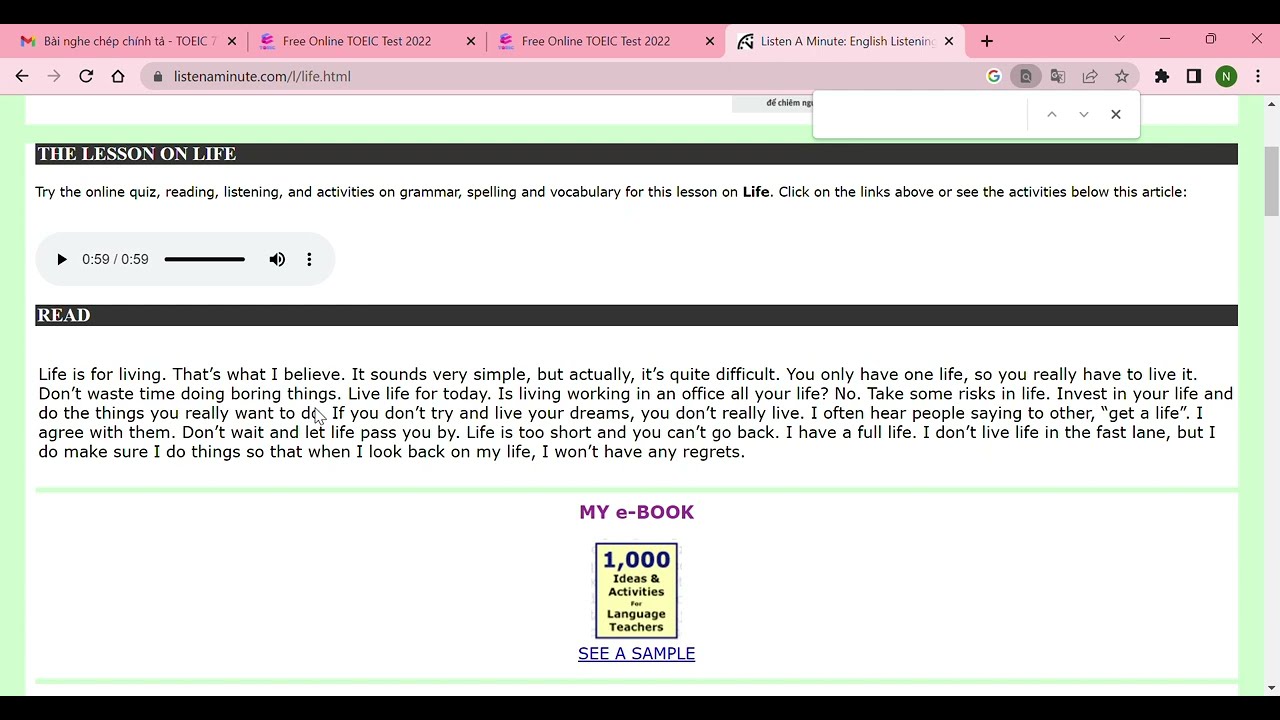The image depicts a screenshot of a computer screen focused on an educational webpage titled "Lesson on Life," hosted on listenaminute.com. At the top of the screen, four browser tabs are visible, with the active tab displaying a lesson aimed at language learners. The primary content includes an invitation to try an online quiz featuring reading, listening, and activities related to grammar, spelling, and vocabulary. A prominent heading "Lesson on Life" is set against a black background with white text, immediately followed by options to engage with various activities through clickable links and a 59-second audio play button symbolized by a speaker icon.

The main passage begins with the text "Life is for living, that's what I believe," and continues to expound on the significance of living life fully, taking risks, and avoiding regrets. This inspirational blurb emphasizes seizing the day and making meaningful choices. Below this passage, there is an advertisement for an e-book titled "A Thousand Ideas and Activities for Language Teachers," with an option to "see a sample." The overall design of the page is simple, mostly in black and white, resembling a standard, unembellished webpage focused on delivering educational content efficiently.